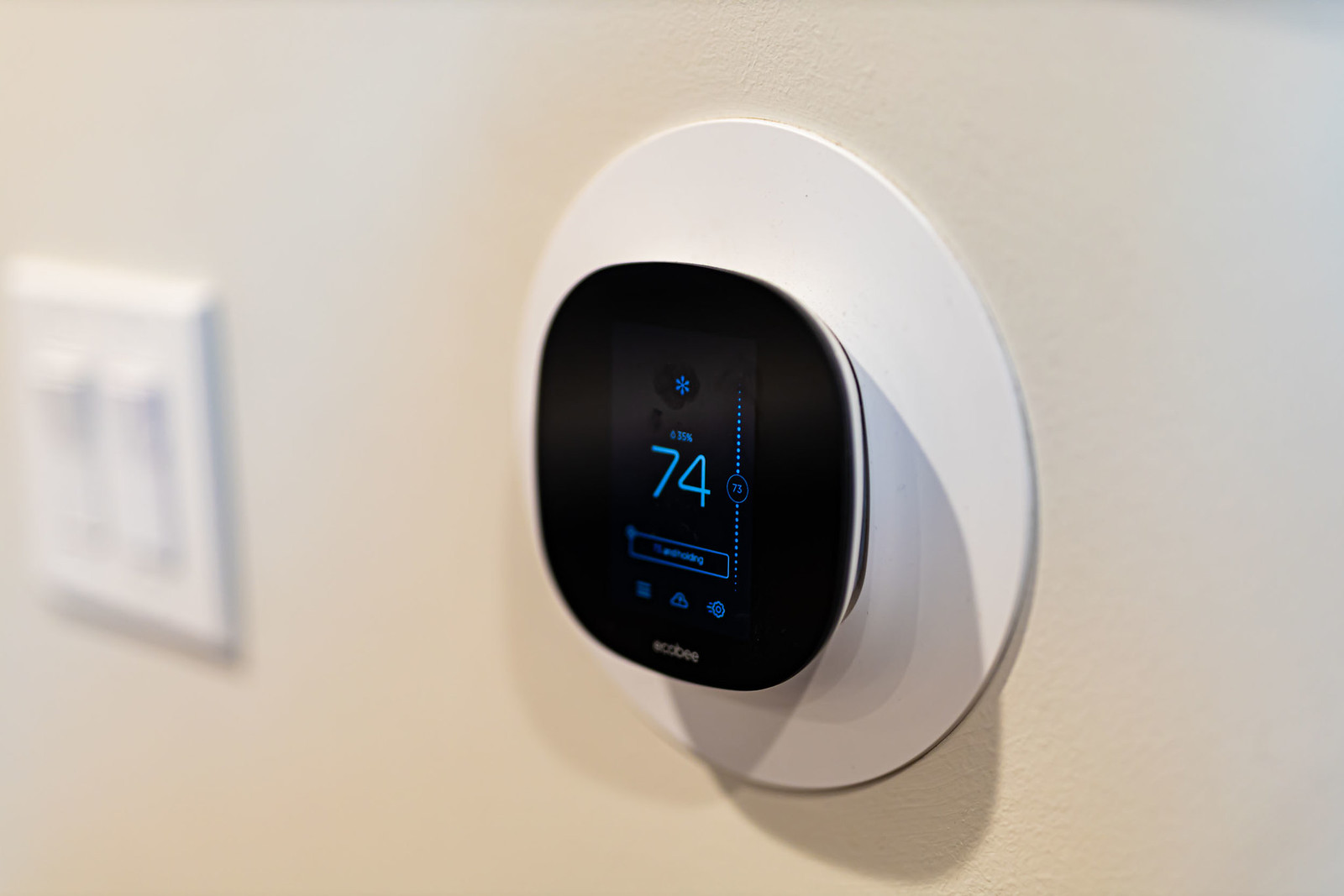The image depicts a digital thermostat mounted on an off-gray wall. A slightly blurred white light switch is visible towards the left side of the photo. The thermostat itself is housed within a circular white mount. Featuring a black digital display, the thermostat shows blue letters and numbers. At the top of the display, a snowflake symbol is prominently visible, indicating cooling mode. Below the symbol, the temperature is set to 74°F. There are also a few additional icons beneath the temperature reading, though they are indistinct due to the distance from which the photo was taken.